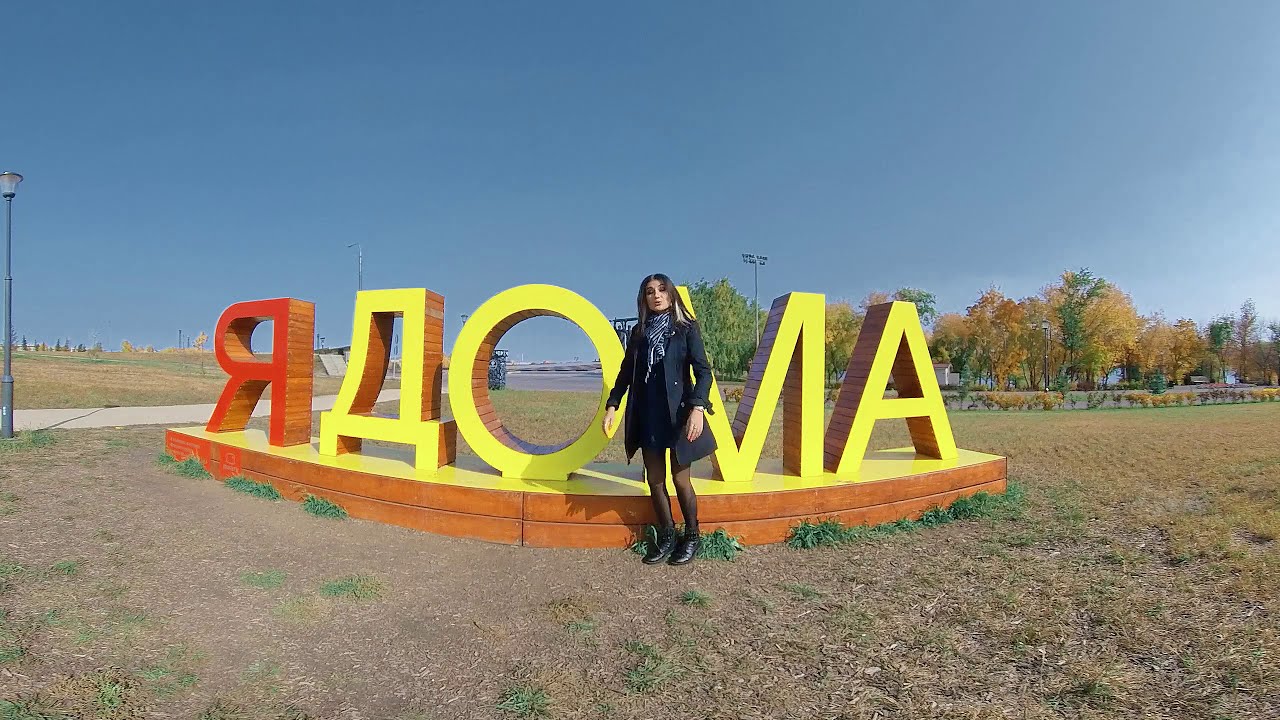This photograph captures an outdoor field featuring a mixture of green and dry brown grass. In the center of the field stands a large concrete platform displaying a vibrant yellow and red text sculpture, possibly in the Russian language. A woman, who appears to be a young, white lady, is positioned directly in front of the statue, facing the camera. She is dressed in a black or dark blue overcoat, a skirt, and black shoes. She accessorizes with a neck scarf and appears to be wearing stockings. Her long, flowing hair, which shows hints of brown and gray, is left open. The background reveals a clear, blue sky, several lampposts, and a collection of trees, along with a faint glimpse of a distant cityscape. The grass in the garden area appears neatly cut. The slightly curved image also suggests a panoramic or wide-angle view.